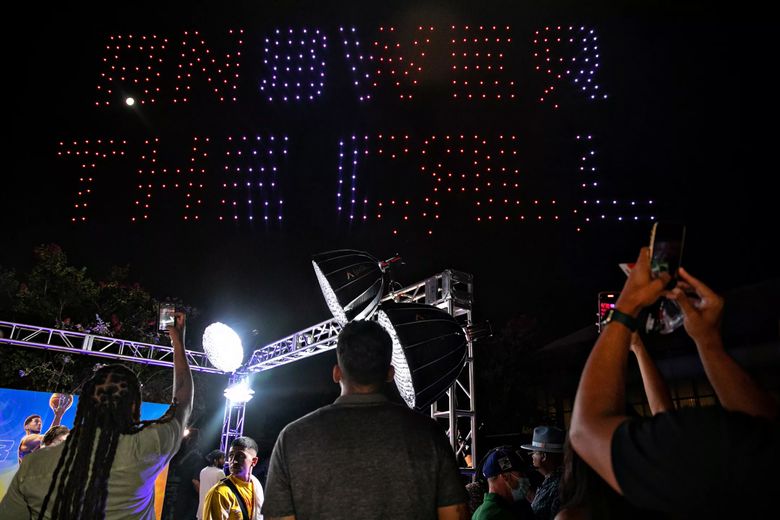This nighttime photograph captures the vibrant atmosphere of an outdoor music festival. Dominating the dark background are illuminated words in white and orangey lights, spelling out "Answer the Call." Beneath this celestial message, a stage is partially visible, framed by intricate metal structures and spotlights.

In the foreground, various people are seen from behind, their identities obscured by the shadows and the angle of the photograph. Among the crowd is a central figure in a gray short-sleeved shirt, facing the sign, and next to him stands a person with black braids in a light-colored shirt, arm raised to capture the moment with a phone. To the right, another individual in a dark shirt also aims a cell phone at the sign, identifiable by the band on their left wrist. Scattered around are more festival-goers, some partially visible, such as a person in a yellow shirt and another wearing a stocking cap.

The stage’s metal pillars and bars cut through the scene, supporting three prominent spotlights. These elements, along with the enthralled crowd and their glowing devices, perfectly encapsulate the communal joy and awe inspired by the festival ambiance.